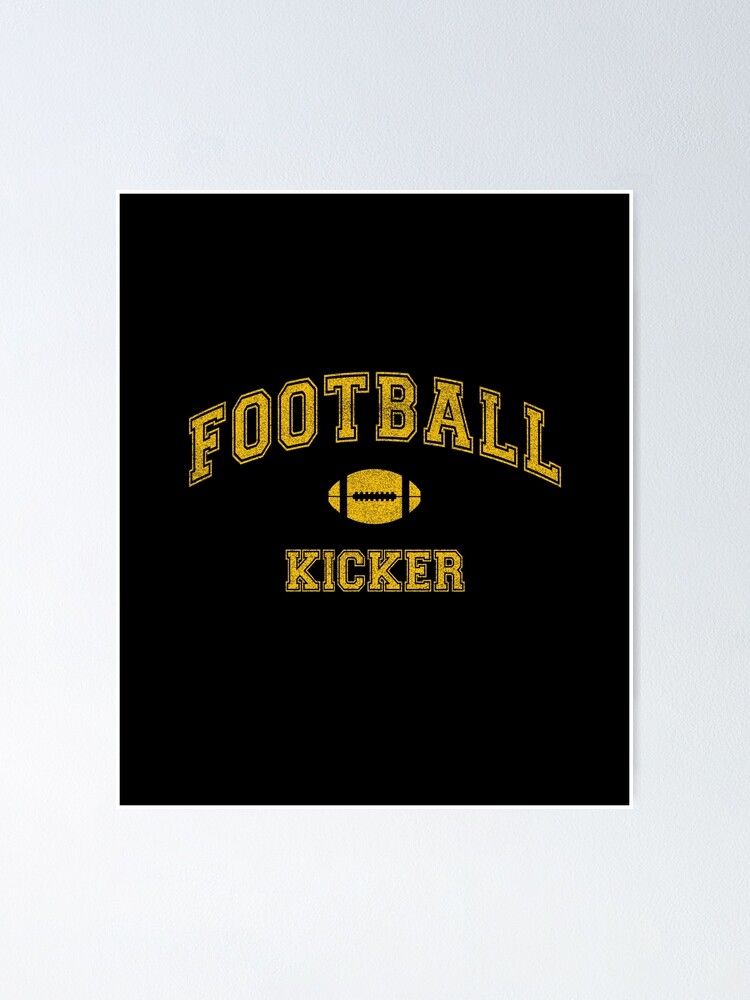The image features a striking print positioned against a slightly textured white background. The print itself, which is slightly longer than it is wide, is set within a thin white perimeter and filled with a solid black backdrop. At the center of the print, the phrase "FOOTBALL KICKER" is prominently displayed. The word "FOOTBALL" appears in a larger, curved sports-style font reminiscent of jersey lettering, with "KICKER" positioned beneath it in a smaller, matching font. Separating the two words is an animated depiction of a football. The text and football both sport a bold yellow hue with black detailing, enhancing their visibility against the dark background. This clean and impactful design underscores the football-themed message with clear, blocky lettering commonly associated with sports aesthetics.